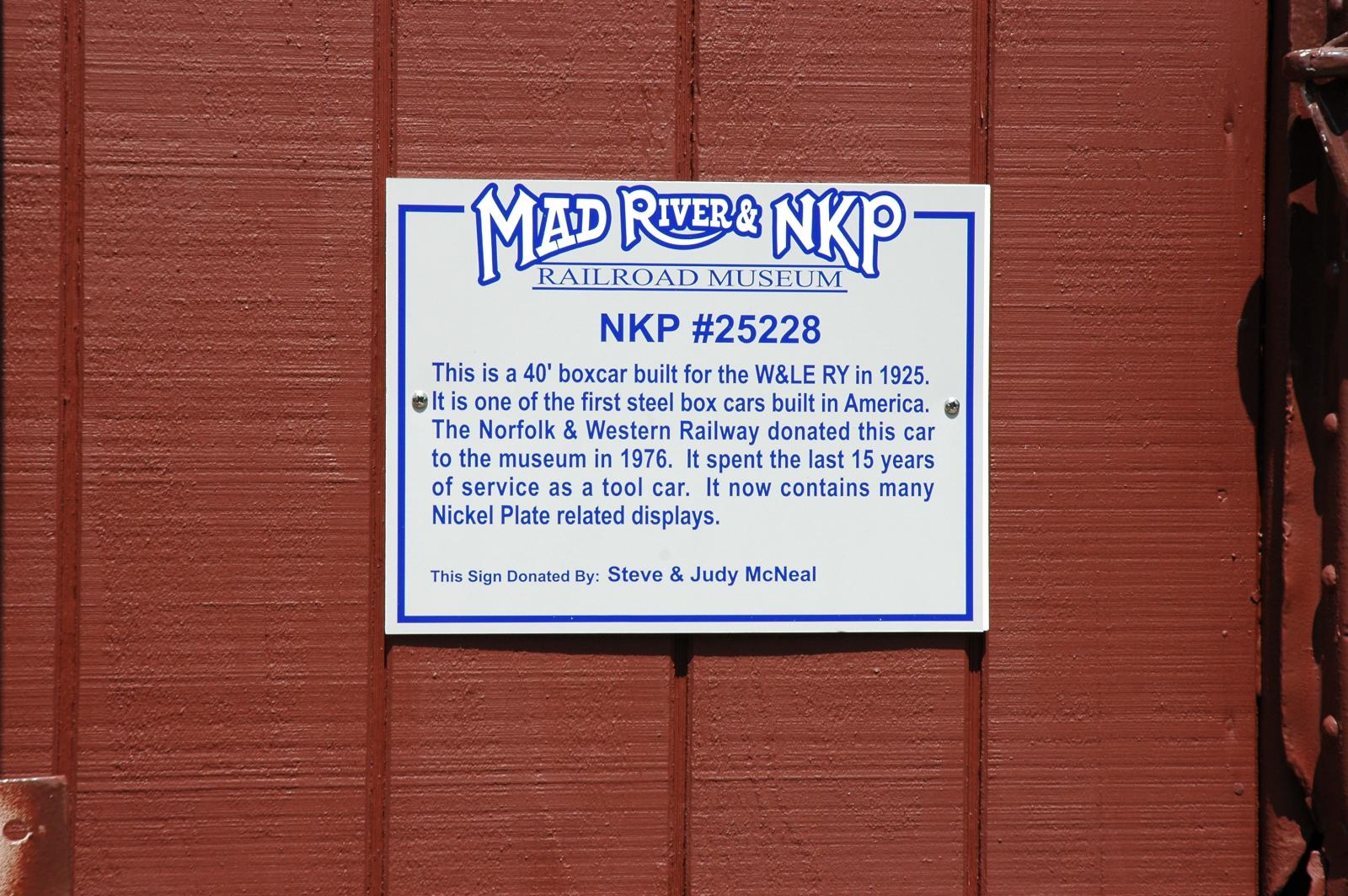The photo depicts a descriptive white sign with blue borders set against a vertically slatted red wooden background with a rust-like hue. The sign prominently features the name "Mad River and NKP Railroad Museum" at the top, followed by "NKP number 25228." Below, in blue text, it states that the displayed item is a 40-foot boxcar built for the W&LERY in 1925, noted as one of the first steel boxcars made in America. The Norfolk and Western Railway donated this boxcar to the museum in 1976, after it had served its final 15 years as a tool car. Now, it houses numerous Nickel Plate-related displays. Additionally, there's a mention in the lower-left corner that the sign itself was donated by Steve and Judy McNeil.